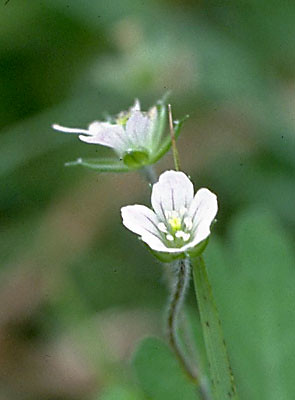The image is a rectangular outdoor photograph featuring two delicate white flowers as the primary focus. The background is predominantly a green blur, hinting at various plants and leaves, but remains out of focus to maintain emphasis on the blooms. The flowers emerge from green stems adorned with fine white fuzz, resembling a soft, feather-like texture. Each flower has white petals accented with subtle green lines and tiny white and yellow buds at the center, presenting a detailed and visually captivating composition amidst the blurred natural backdrop.